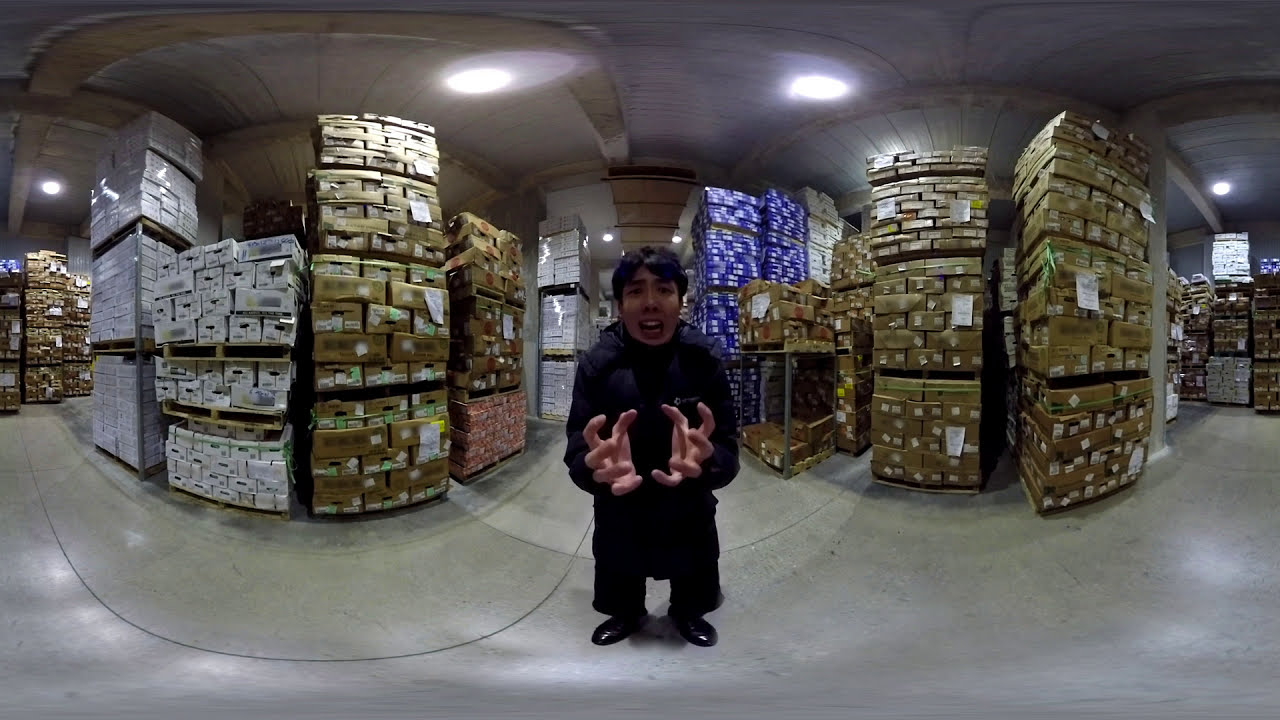In this dimly lit warehouse with fluorescent lights on the ceiling, numerous pallets stacked with brown, white, blue, and a few red boxes extend around the area, some piled as high as the ceiling. The smooth, light concrete floor reflects the industrial setting's vastness. At the center, a young man dressed entirely in black—jacket, pants, and shoes—dominates the scene with a grimace of distress on his face, his mouth slightly open. His medium-length black hair frames his expression of pain or fear, while his hands are stretched out in front of him, fingers curled as though grasping for something unseen. The image appears manipulated, with visible curves on the sides and blurred-out labels on many of the boxes, enhancing its eerie, surreal quality.